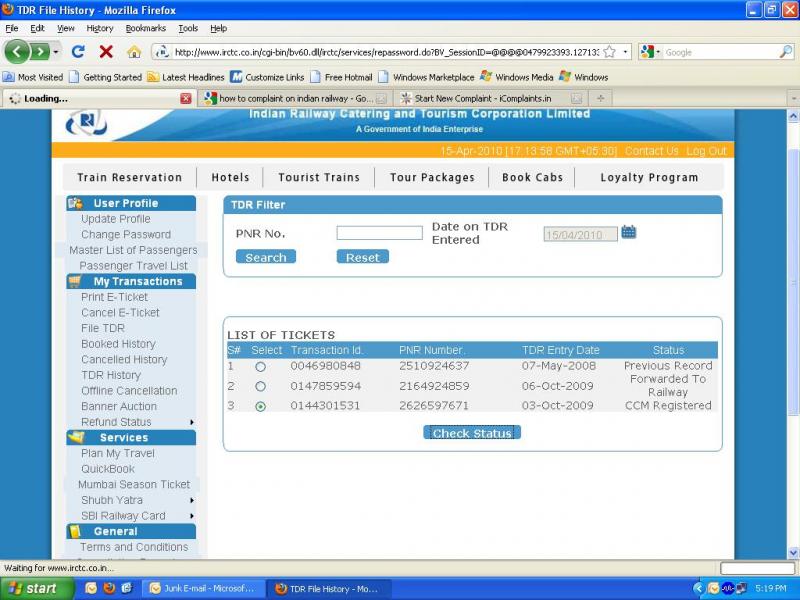Screenshot of an old computer interface, possibly running Windows 7. The top bar is blue and features a dated Firefox icon next to the label "TDR File History". To the right, the minimize, maximize, and close buttons are visible. Just below, the traditional menu items—File, Edit, View, History, Bookmarks, Tools, Help—are laid out, followed by navigation buttons (back, forward, refresh, etc.), an address bar, and a Google search bar.

Below the navigation area, there is a row of bookmarks labeled: Most Visited, Getting Started, Latest Headlines, Customized Links, Free Hotmail, Windows Marketplace, Windows Media, and Windows.

The main content displayed is from the Indian Railway Catering and Tourism Corporation (IRCTC), a government of India enterprise. The webpage has a color scheme of blue and orange with a white background. Key menu options include:

- Train Reservation
- Hotels
- Tourist Trains
- Tour Packages
- Book Cabs
- Loyalty Program

The left sidebar provides various user functions:
- User Profile
- Update Profile
- Change Password
- Master List of Passengers
- Passenger Travel List
- My Transactions
- Print Ticket
- Cancel Ticket
- File TDR
- Booked History
- Cancelled History
- TDR History
- Online Cancellation
- Refund Status
- Services
- Plan My Travel
- QuickBook
- Mumbai Season Tickets
- Shubh Yatra
- SPI Railway Card
- General Terms and Conditions

A blue box titled "TDR Filter" contains fields for "PNR Number" and "Date on TDR Entered" with an example entry "15/04/2010" followed by search and reset buttons. Another blue box below is labeled "List of Tickets," showing columns for "S. Number," "Select," "Transaction ID," "PNR Number," "TDR Entry Date," and "Status." Listed are three tickets with various details, including entries from May 7, 2008, October 6, 2009, and October 3, 2009. At the bottom, a blue button labeled "Check Status" is displayed.

The entire interface is framed with typical old Windows iconography at the bottom of the screen.